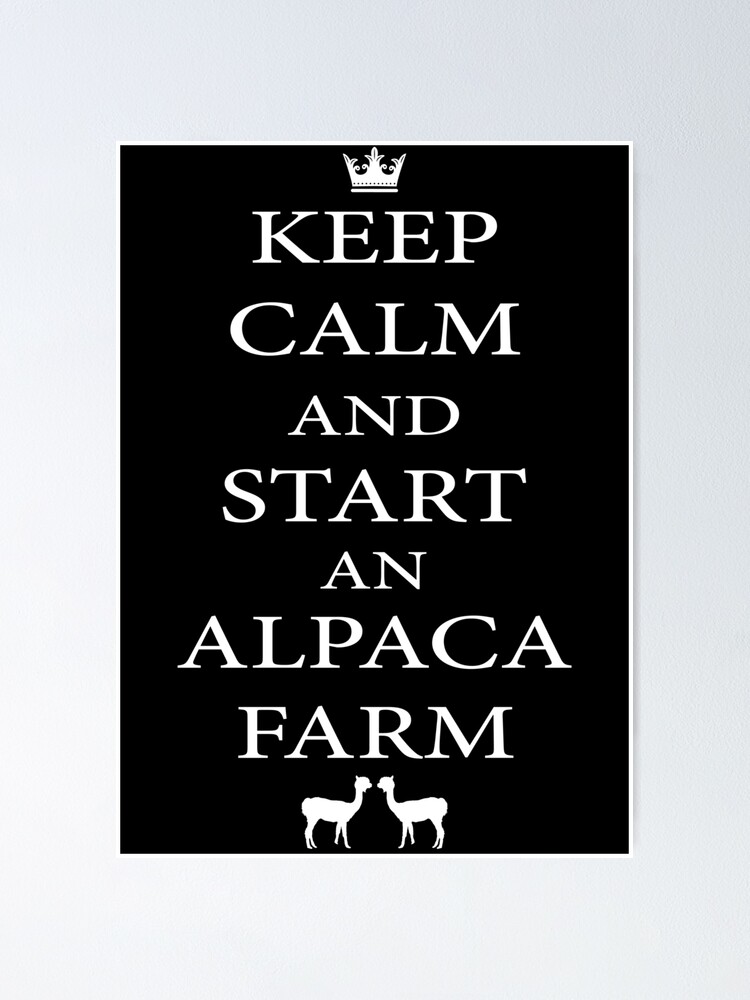The image features a vertical sign set against a light gray wall, framed with a very thin white border. The graphic, centered perfectly both vertically and horizontally, has a black background. At the top of the graphic, there is a white, three-pronged crown adorned with sharp spikes and a small decorative piece at the top center. Below the crown, in all capitalized, serif font white text, the words "KEEP CALM AND START AN ALPACA FARM" are displayed, with "KEEP CALM," "START," and "ALPACA FARM" being the same size, and "AND" and "AN" slightly smaller. At the bottom of the graphic, two white outlined alpacas facing each other are depicted, mirroring each other with minimal detail.